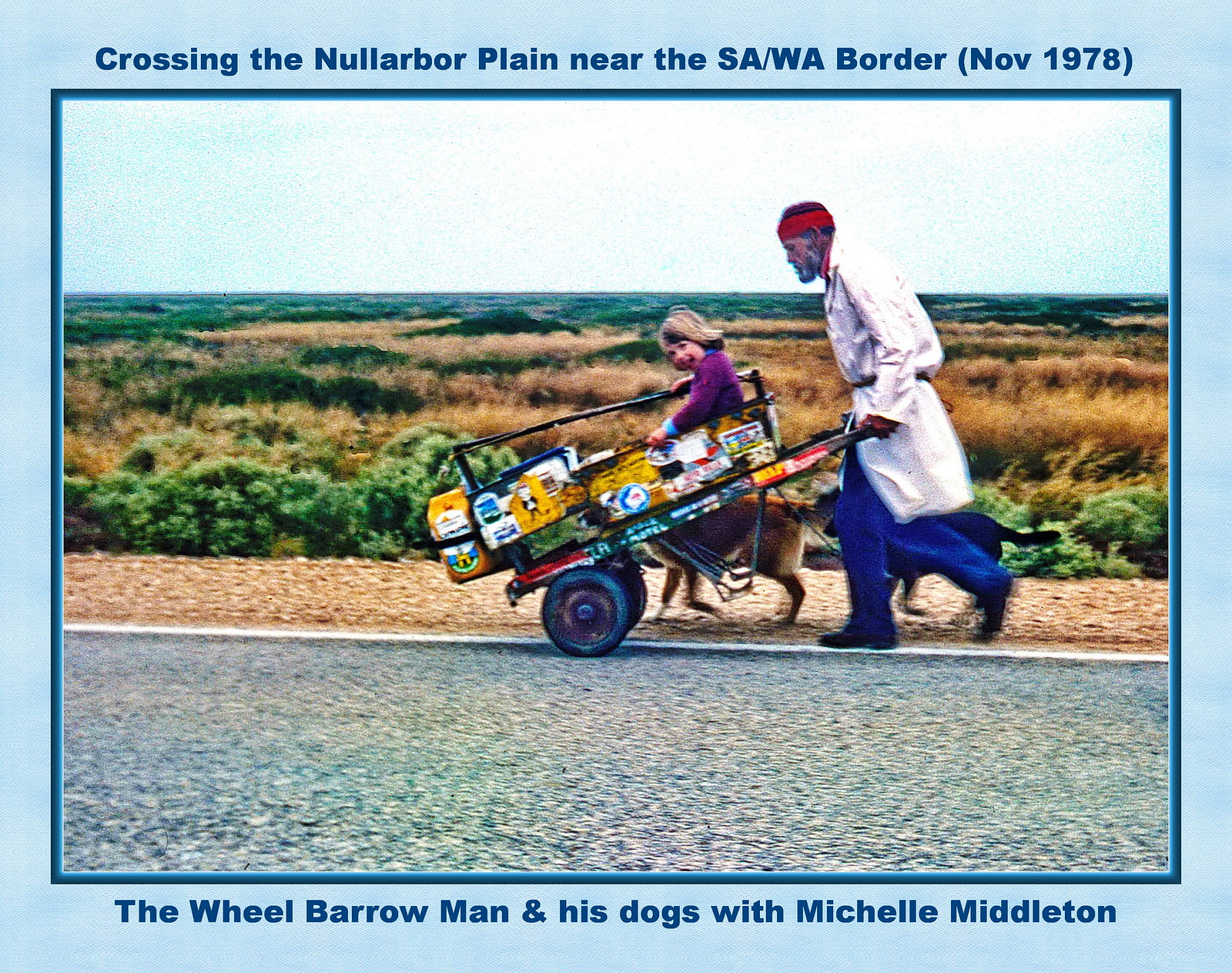This photograph captures a man pushing a unique wheelbarrow along the side of a road. The man is dressed in a white suit that falls just below his knees, blue pants, black shoes, and a red bandana tied around his head. He sports a full beard with hints of gray. The wheelbarrow itself is adorned with various stickers and features two front tires and a metal round barrier. Inside this barrier, a child with blonde hair, dressed in a purple shirt, sits facing back towards the camera. A brown dog with white patches under its stomach and on the back of its legs trots alongside them. The scene is set on a gray asphalt road marked with a white line, bordered by a strip of light brown gravel and lush vegetation comprising dark green plants and some yellowing grass. Surrounding the image is a light blue border. Text above the photograph reads, “Crossing the Nullarbor Plain near the SA/WA border in November 1978,” while the caption at the bottom states, “A wheelbarrow man and his dogs with Michelle Middleton.”